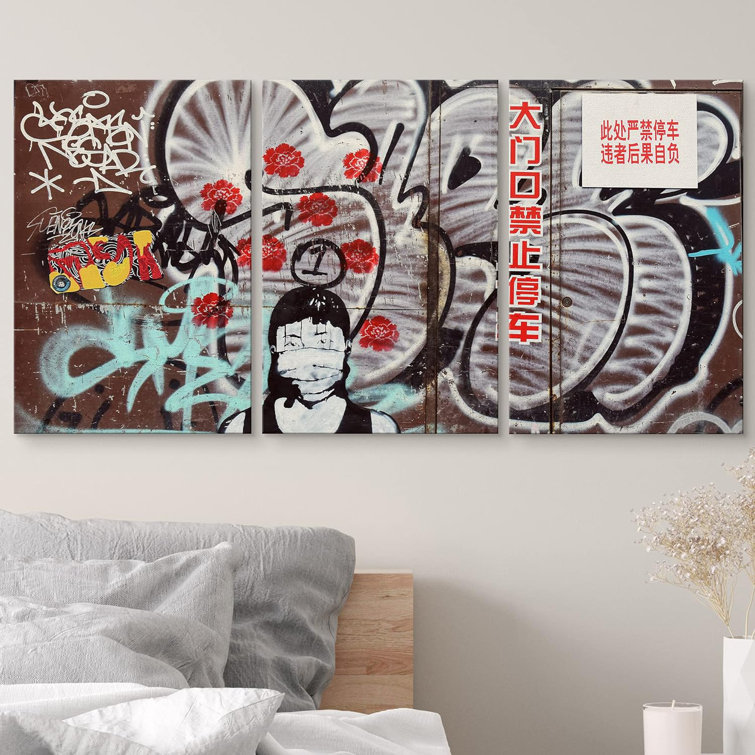This photograph captures a cozy corner of a bedroom, with a strong focus on the artistic elements above the bed. The bed itself is anchored by a wooden headboard, partially visible beneath an array of pillows. At the bottom left, two white pillows are tucked in front of a light gray pillow, which is propped up in front of a dark gray pillow nestled against the headboard. To the right of this arrangement, a white candle stands beside a taller white candle, accompanied by a house plant that adds a touch of greenery.

The gray-colored wall behind the bed provides a neutral backdrop for a striking piece of artwork that spans the upper portion of the image. This piece appears to be a collage of three segments, exuding a graffiti-like aesthetic with vibrant colors and intricate designs. A prominent vertical strip of red Asian characters runs down one part of the artwork, while adjacent to it, another set of similar characters is etched against a white background. The lower section of the artwork features the face and upper torso of a young girl, possibly Asian, wearing a mask. This art piece, rich in red, white, and yellow hues against a brown background, infuses an edgy, urban feel into the otherwise serene bedroom setting.